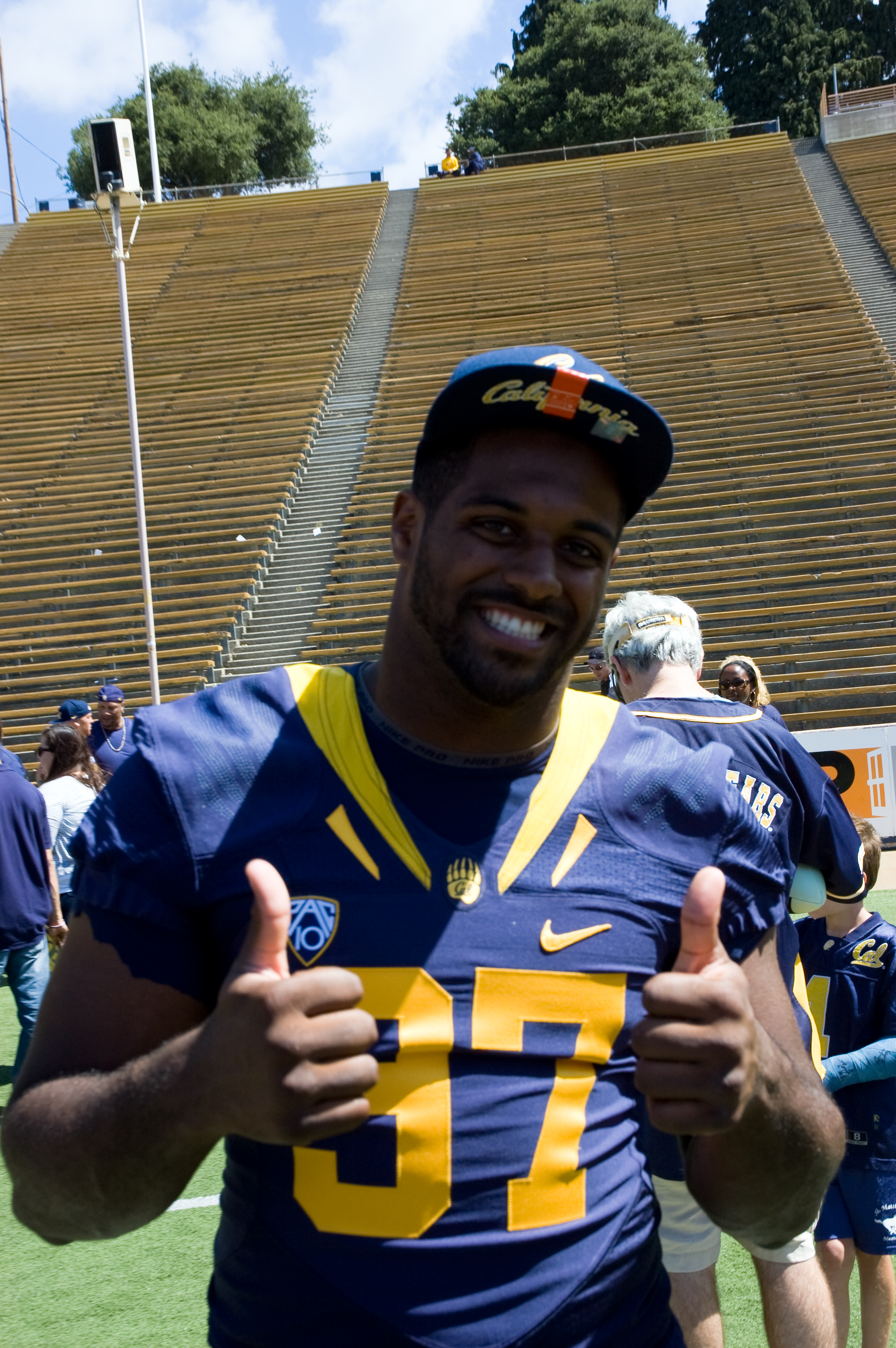A wide-angle photograph taken from the bottom of an empty stadium showcases rows of vacant seats cascading upwards to the top, where the tops of green trees are just visible. In the foreground, a football player stands prominently with his thumbs up. He is an African-American man wearing a dark blue football jersey adorned with the number 87, the Nike logo, and the text "Pack 10" above the numeral. Accompanying him, slightly behind and to the side, is a coach with gray hair and a black woman who appears to be looking downward. The clarity of the deserted stadium seats against the lively expressions and gestures of the individuals in the foreground creates a striking and dynamic visual contrast.